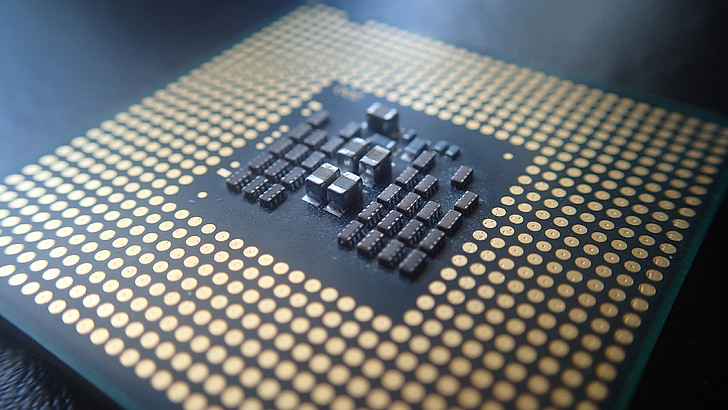The image features a close-up of a circuit board or microchip, distinguished by its green outer edge and square shape. Dominating the periphery are numerous metallic, gold-like dots arranged in an ordered array, estimated to be around 200 in total, forming nine distinct rows. The center of the board is a contrasting black area populated with various components, chips, and transistors, suggestive of a space meant for significant electronic elements such as a processor. The setup sits on a textured, dark gray and black surface, with faint traces of smoke or steam in the background, lending an industrial, in-progress feel to the image.